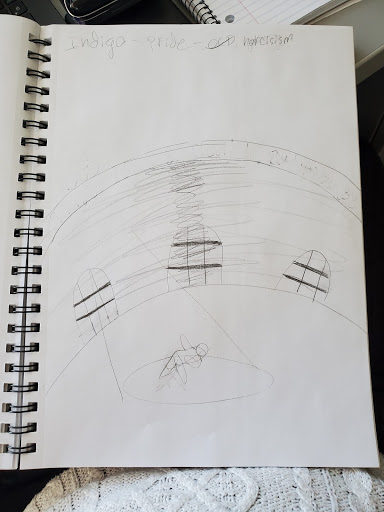The photograph captures a sketchpad with a metal ring binding, placed on a desk. The sketchpad displays artistic handwriting at the top that reads "Indigo Pride Narcissism," with the word "OCD" crossed out. The drawing features a figure, possibly dancing or skating, illuminated by a spotlight. Surrounding the figure is a circular structure with three arched windows, each bearing a tic-tac-toe-like frame design. The sketch appears to be rendered in either pencil or fine grey crayon. There is a secondary notebook visible in the top right corner of the image, and in the foreground, a white textured woolly jumper or blanket is partially visible. The drawing has an amateurish, traced quality, emphasizing simplicity and expressiveness.